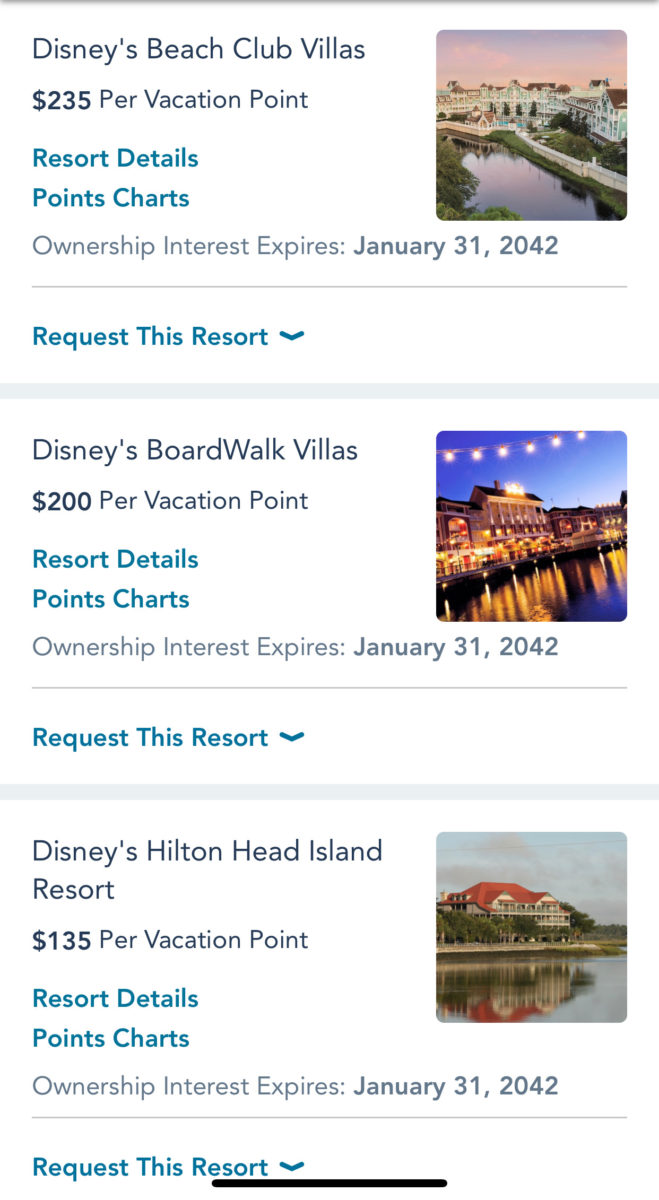### Detailed Descriptive Caption

This image showcases a clean and simple layout from an e-commerce website, specifically highlighting three separate listings for Disney vacation resorts. The background is predominantly white, with clear delineations made by thin gray and green lines, which segment each listing like borders.

The top listing on the page features "Disney's Beach Club Villas." The structure is as follows:
- **Left Side:** 
  - At the top, there is a thin gray border line.
  - Directly below, the title "Disney's Beach Club Villas" is prominently displayed.
  - Underneath the title, it states "235 per vacation point" indicating the cost.
  - Following the cost, there are interactive green text links labeled "Resort Details" and "Points Chart."
  - At the very bottom, it mentions, "Ownership interest expires January 31, 2042."
  - The segment concludes with a gray line inscribed with “Request This Resort,” followed by another green border line.
- **Right Side:** 
  - Accompanying the textual information is a small representative photo of the resort.

Directly below, two additional listings follow the same format:
- **Second Listing:** 
  - Titled "Disney's Boardwalk Villas." 
  - Priced at "200 per vacation point."
  - Includes green clickable links for "Resort Details" and "Points Chart."
  - Indicates the ownership expiration date.
  - Features the same end-of-segment lines.
  - Accompanied by a photo of "Disney's Boardwalk Villas."

- **Third Listing:** 
  - Labeled "Disney's Hilton Head Island Resort."
  - Listed at "135 per vacation point."
  - Features clickable green text links for detailed resort information and points chart.
  - Includes ownership expiration details.
  - Concludes with the same delineation and visual format as previous listings.
  - Displays a relevant photo of "Disney's Hilton Head Island Resort."

The entire page is neatly organized with a final black line at the bottom, indicating the end of the listings.